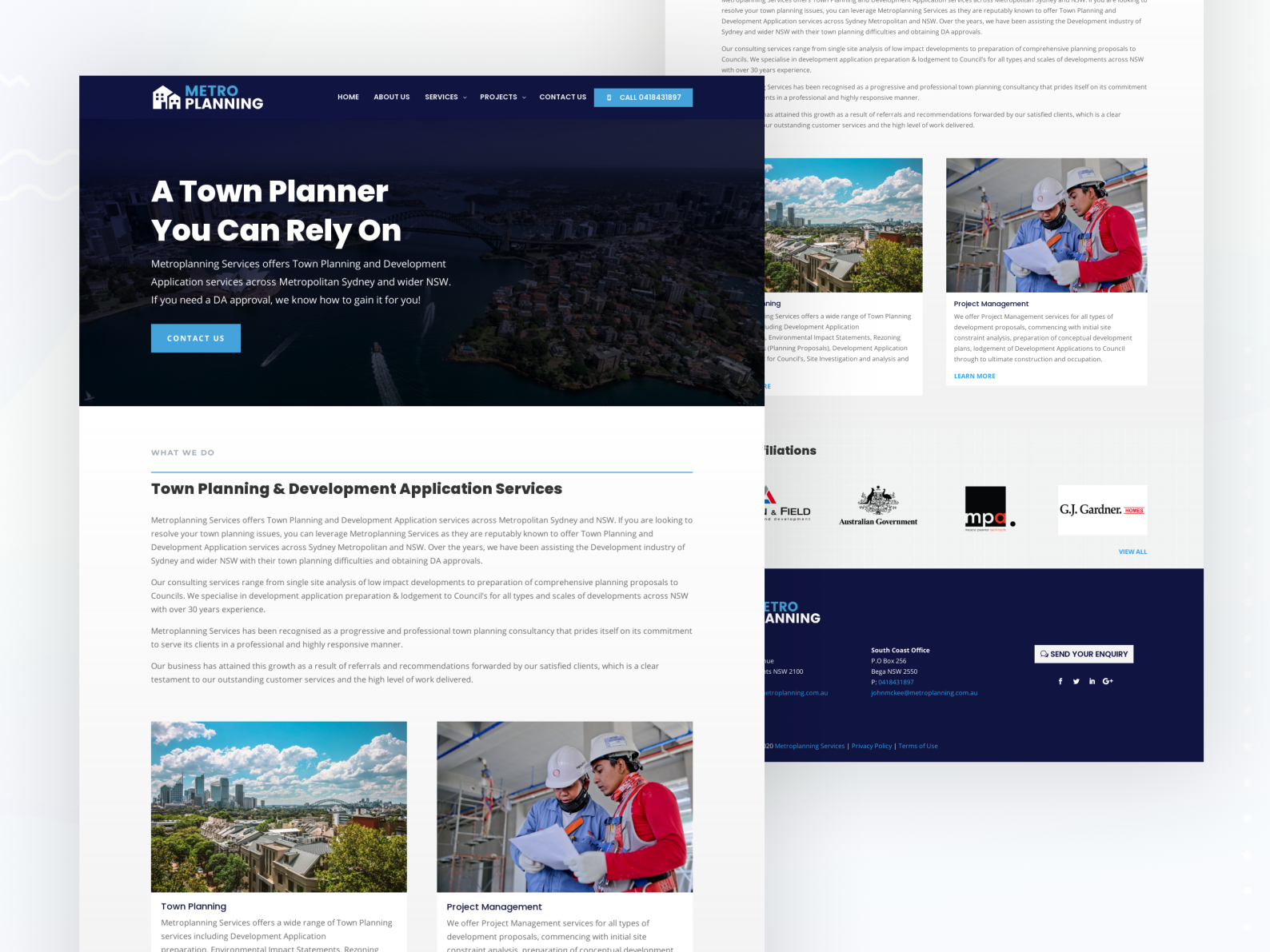The image depicts two sections of a web page overlaid on a light gray background, each casting a faint medium gray shadow. The upper right section showcases a photograph of a dense city by a river, darkened with a deep blue shade in the top left corner. In this section, a logo featuring two overlapping white houses—with the larger house on the left—sits prominently. To the right of this logo, the words "Metro" in blue and "Planning" in white are displayed. Further right, white text reads "Home," "About Us," "Services" with a white arrow pointing downwards, "Projects" with another white arrow pointing downwards, and "Contact Us." 

Adjacent to this text is a bright blue button featuring a white cell phone icon on the left and the words "Call 0418 431 897" on the right. Below this, large white text asserts, "A town planner you can rely on." Beneath this phrase, smaller white text reads: "Metro Planning Services offers town planning and development application services across Metropolitan City and wider NSW. If you need a DA approval, we know how to gain it for you." At the bottom of this section, on the left, there is another bright blue button with the text "Contact Us" in white.

The lower left section of the web page continues with a white background and additional text.